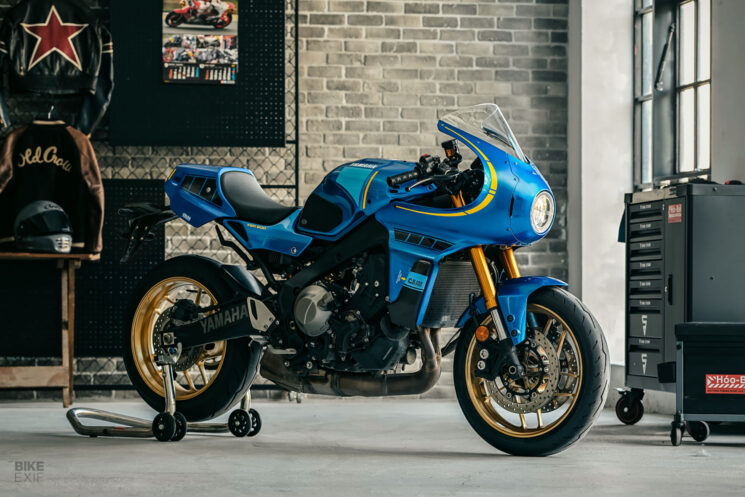The image features a striking Yamaha motorcycle with a shiny blue body and gold accents, set indoors against a background with an industrial aesthetic. The front of the motorcycle is turned towards the right side of the image, revealing additional details such as a pair of stabilizing training wheels connected by a loop on the back wheel to prevent it from tipping over. In the room, the right-hand side is home to two gray tool cabinets on wheels, one larger with multiple drawers and a smaller one beside it. The backdrop features an exposed brick wall adorned with various items. On the left-hand side, there's a black and brown jacket hanging above a shelf holding a gray helmet, with another jacket featuring a red star on its back hanging nearby. Additionally, the brick wall is decorated with posters of motorcycles, a lattice-type bulletin board displaying pictures and memorabilia, highlighting the room’s garage-like atmosphere.